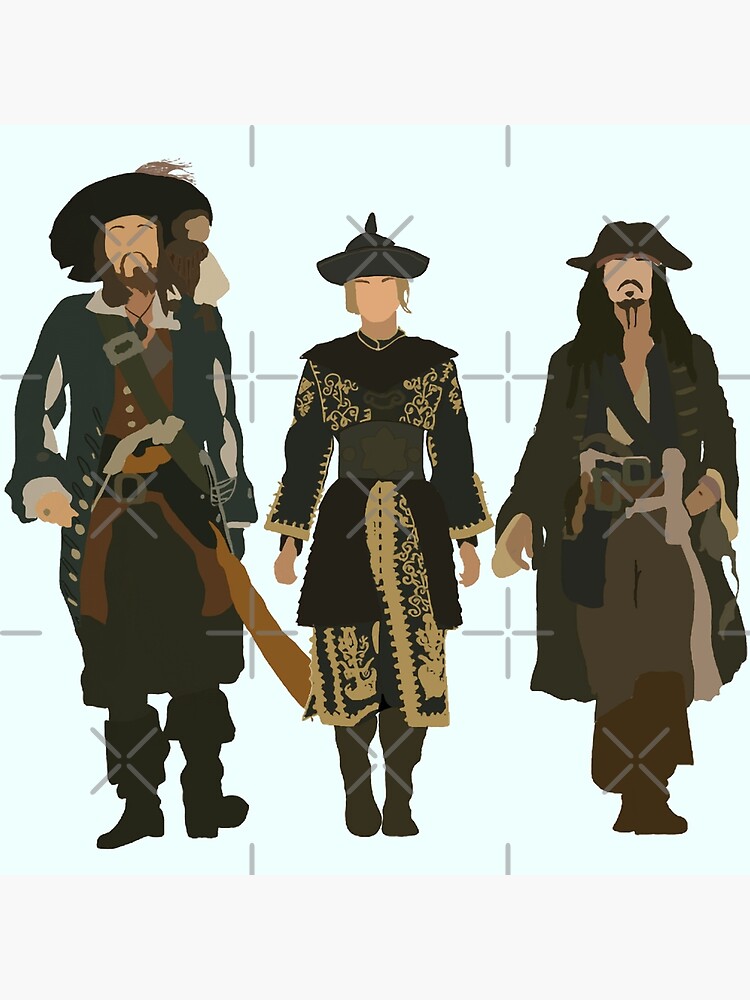This detailed image is a watercolor painting set against a light blue background and features three men dressed in old-timey, black, swashbuckling clothing reminiscent of pirates or musketeers. The men, depicted in Latin American styled attire complete with hats adorned with X's, stand side by side as if walking toward the viewer. Each man's outfit includes buttoned coats and various distinguishable accessories; one appears to have something like a gun hanging at their side. Despite having detailed facial hair—mustaches and goatees—their facial features are notably missing, lacking eyes, noses, and mouths. A prominent cross-shaped design, along with a symmetrical gray tic-tac-toe grid pattern, overlays the image, adding an intriguing, almost heads-up display quality to this distinctive artwork.